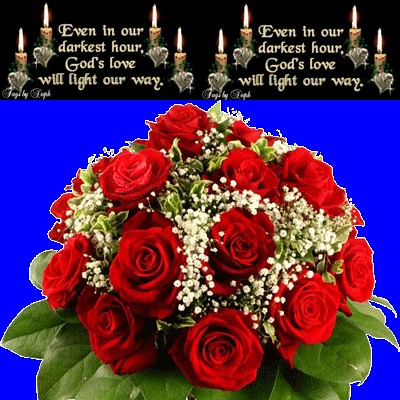The image features a digitally created graphic with a vibrant blue background. At the center, a bouquet of approximately a dozen red roses is prominently displayed, enhanced by sprigs of green leaves and delicate clusters of baby's breath white flowers. Above this floral arrangement, a religious message in gold text reads, "Even in our darkest hour, God's love will light our way," a phrase that is repeated twice. This text is flanked by eight lit candles—four on the left and four on the right—set against a contrasting black background. The candles and the text appear mirrored on either side, creating a symmetrical design reminiscent of something one might find in a sentimental social media post by a grandmother.